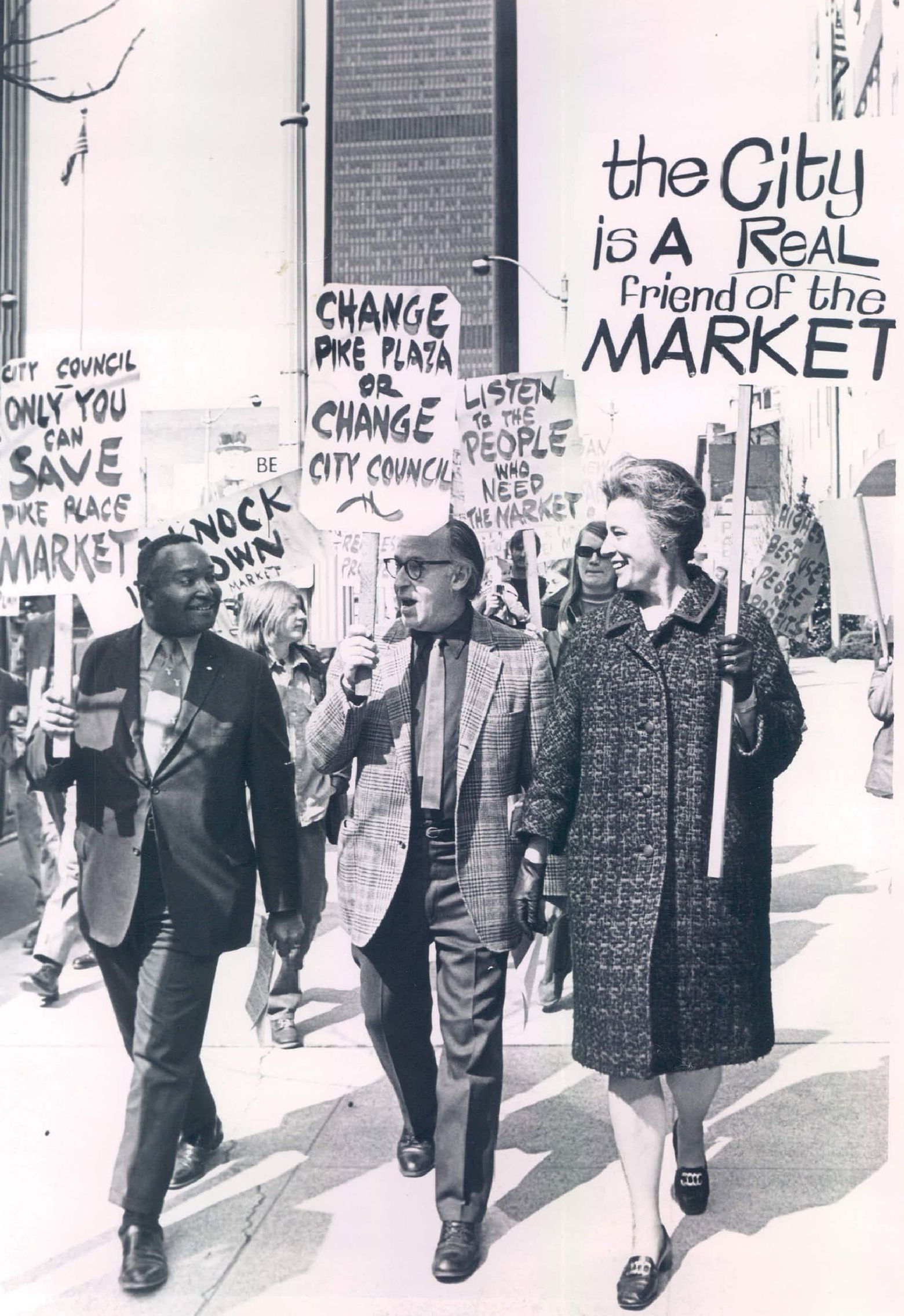The image is an old black-and-white photograph, likely from the 1970s or 1980s, depicting a protest. It has been given a pale pink tone in certain areas, adding a subtle color accent to the otherwise monochromatic scene. The picture is about six inches high and four inches wide, and it captures people marching down a street on a pale pink and light gray stone sidewalk.

In the foreground on the right-hand side, there is a Caucasian woman wearing a long, thick wool overcoat and black gloves, with medium-length helmet-style hair. She holds a sign with black print that reads, "The city is a real friend of the market," and the sign has a slight pink hue. 

To her left and slightly behind her is a Caucasian man dressed in a suit and tie, holding a sign that says, "Change Pike Plaza or change City Council." Near him is another gentleman, also wearing a suit and tie, with short hair and of African descent. He carries a sign that states, "City Council, only you can save Pike Place Market." 

In the background, amid the protesting crowd, additional signs are visible. One partially obscured sign reads, "Knock down," suggesting perhaps "Knock down the market." The protesters march in front of a large, indistinct building that looms in the background against a bright sky.

The overall scene reflects a spirited protest aimed at urging the City Council to take action regarding Pike Place Market, capturing both the urgency and solidarity of the moment.